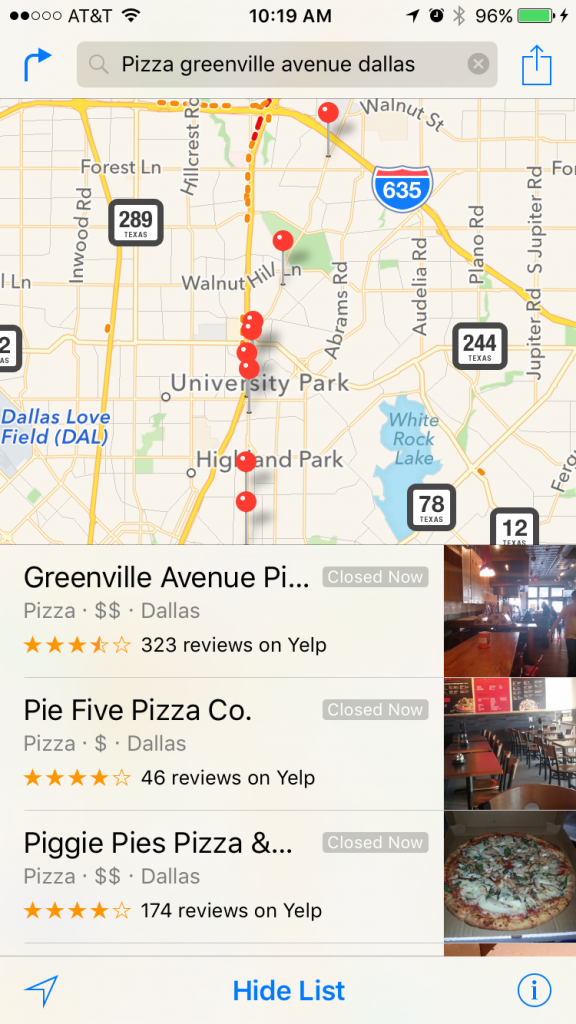Here is a detailed and cleaned-up caption for the image:

---

This is a screenshot taken from a mobile device displaying various details. In the top-left corner, the device shows it's connected to the AT&T network with two out of five cell bars. The Wi-Fi signal is full. The time displayed at the top center is 10:19 a.m. To the right, there are icons indicating an active alarm clock, Bluetooth being enabled, and the battery at 96% charge, with a black lightning bolt symbol indicating that the phone is currently charging.

The main display showcases a map application in use. The user has searched for "Pizza Greenville Avenue in Dallas." The map itself has a yellowish hue with yellow lines representing the roads. Red pin markers indicate specific locations. Below the map, there is a list of pizza places along Greenville Avenue: Greenville Avenue Pizza, Pie Five Pizza Co, and Piggy Pie's Pizza. All three establishments are currently closed.

Each restaurant listing includes reviews and star ratings. At the bottom left of the list, there is an option to hide it, and in the bottom right corner, there is an information button.

---